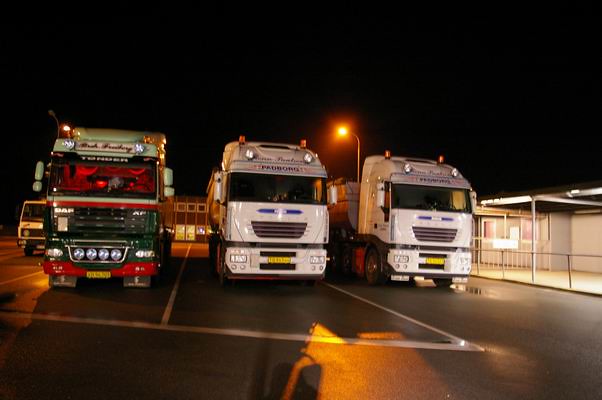The nighttime image captures a scene with a deep black sky providing a stark backdrop to three prominently placed trucks. The focus is on these trucks, arranged side by side on a wet, well-maintained tarmac, possibly a parking area with white lines marking the bays. The two trucks in the middle and on the right are identical, sporting white with light blue accents and yellow license plates, signifying they might belong to the same fleet. The truck on the left stands out with a distinctive light green and red color scheme and also has a yellow license plate. A fourth truck is partially visible in the background behind the green truck.

In addition to the trucks, the image features a neat and uncluttered building to the right, adorned with a railing around its covered patio area. Another notable element is a lamppost in the background, emitting a bright orange light that casts an orange corona, possibly mistaken for the moon. The cement beneath the trucks appears wet, hinting it might have rained recently, with a noticeable puddle near the truck on the far right. The scene suggests a commercial business or service area where the trucks might have stopped for the night.